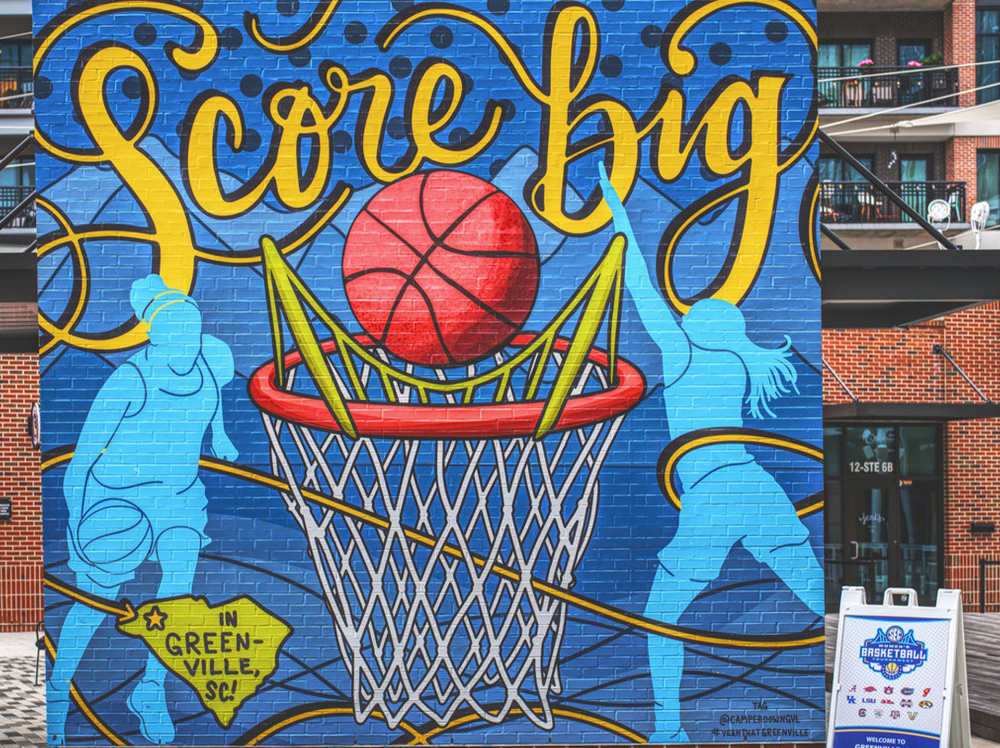This is an image in landscape orientation of a painted mural on a brick wall, located in front of a brick apartment building with visible balconies. The mural, covering nearly the entire height of the image from the left edge to about two-thirds across, features a vivid blue background. At the top of the mural, in yellow script with a black drop shadow, the text "SCORE BIG" stands out prominently. Central to the mural is a red basketball hoop, depicted without a backboard, with an orange basketball suspended above it as if about to fall through the net. Flanking the hoop are teal blue silhouettes of female basketball players; the one on the left is dribbling a ball, while the one on the right appears to be leaping to block a shot. In the bottom left corner is a yellow outline of the state of South Carolina, marked with a black star in the top left and inscribed with black text that reads "IN GREENVILLE SC!" On the bottom right, there is a white standing tent sign, promoting an event, set against the backdrop of the brick apartment building behind.